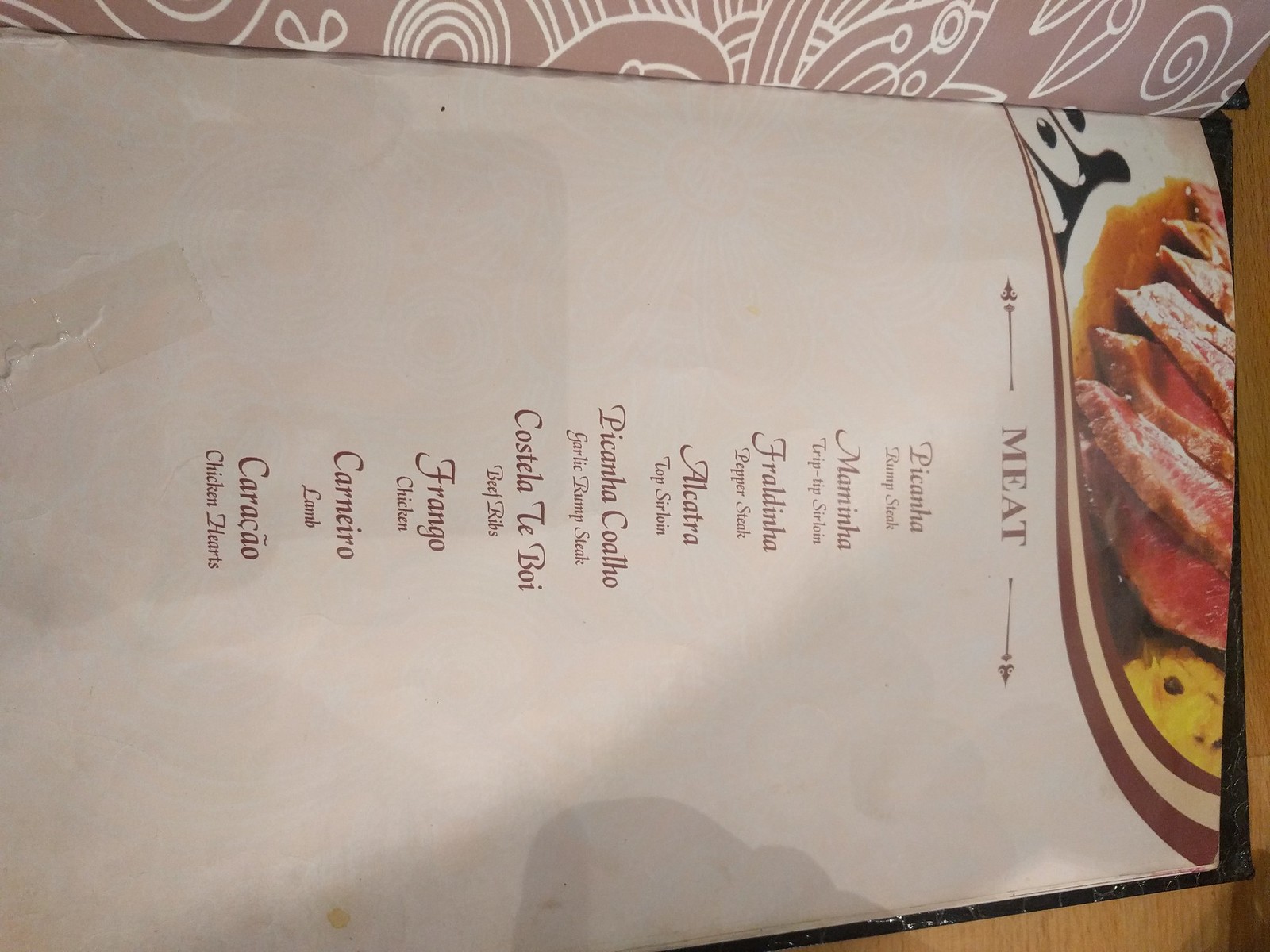The image depicts a scruffy, landscape-oriented menu that requires turning one's head 45 degrees to the right for proper viewing. The condition of the menu shows some wear and tear, with a taped-up portion and possible greasy stains, though it might just be shadows creating that effect. On the right side, there's a partial image of a plate showing meat topped with sauce and accompanied by what appears to be mashed potatoes.

At the top center of the menu, the heading "MEAT" is prominently displayed in a fancy font, flanked by arrows pointing left and right. The menu lists various meats in the middle of the page, also aligned centrally, and includes items such as:

- Picanha (rump steak)
- Mamina (also referred to as trip tip sirloin)
- Top sirloin
- Garlic rump steak
- Beef ribs
- Chicken
- Lamb
- Chicken hearts
- Frango (chicken)
- Alcatra (top sirloin)

The menu is notable for its lack of pricing and detailed descriptions for each item.